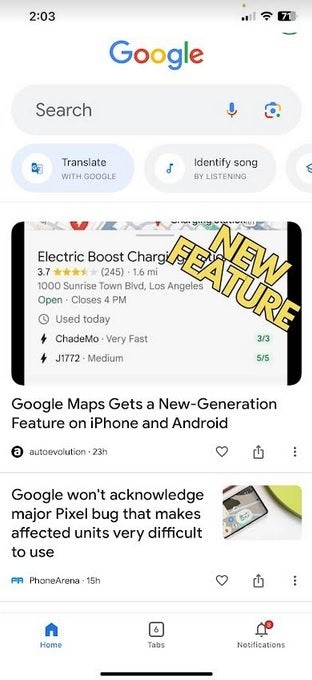This screenshot, taken on a mobile phone at 2:03, captures a Google search page. The mobile interface shows a 71% battery life, strong cell signal, and active Wi-Fi connection in the top-right corner. The upper portion of the screenshot features the iconic Google logo followed by the Google search bar. On the left below the search bar is a button labeled "Translate with Google," while to its right is a button for "Identify Song."

The primary search result highlighted involves a Google Maps announcement regarding a new feature available on both iPhone and Android platforms. Just above this text, there's an image labeled "Electrical Boost," likely related to charging, accompanied by the location's address and star rating. In the image's top-right corner, a yellow text banner reads "New Feature." Further down, another headline states, "Google won't acknowledge major Pixel bug that makes affected units very difficult to use," with an accompanying image of a Google Pixel phone located to the right.